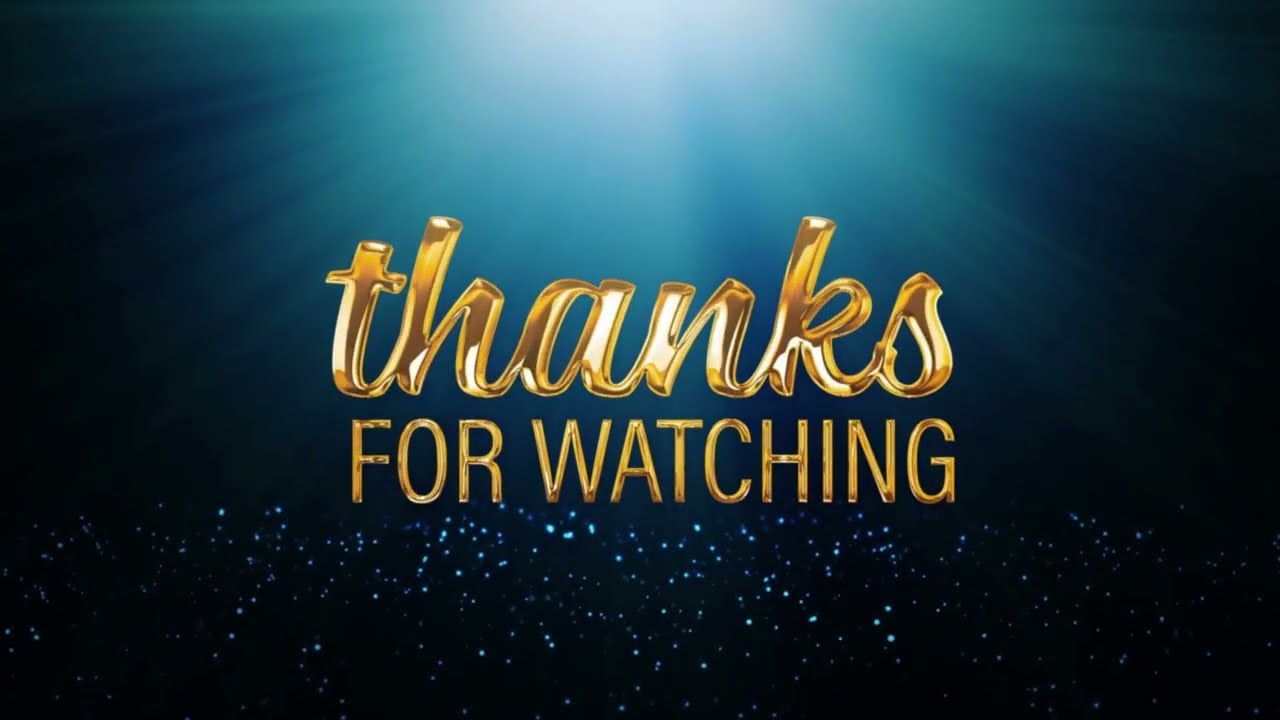The image is a digitally illustrated announcement with a predominantly blue background that mimics an underwater scene or a night sky. A radiant light source shines from above, making the center a lighter blue that gradually fades to a deep, nearly black shade towards the edges. The focal point of the design is the gold, shiny text. The word "THANKS," written in cursive and featuring a 3D effect, is centered in the upper portion of the image. Below it, in a smaller sans-serif, all-caps font, are the words "FOR WATCHING." Beneath this text are sparkles or bubbles that add a glittery effect to the bottom section, enhancing the overall ethereal and immersive feel of the scene.